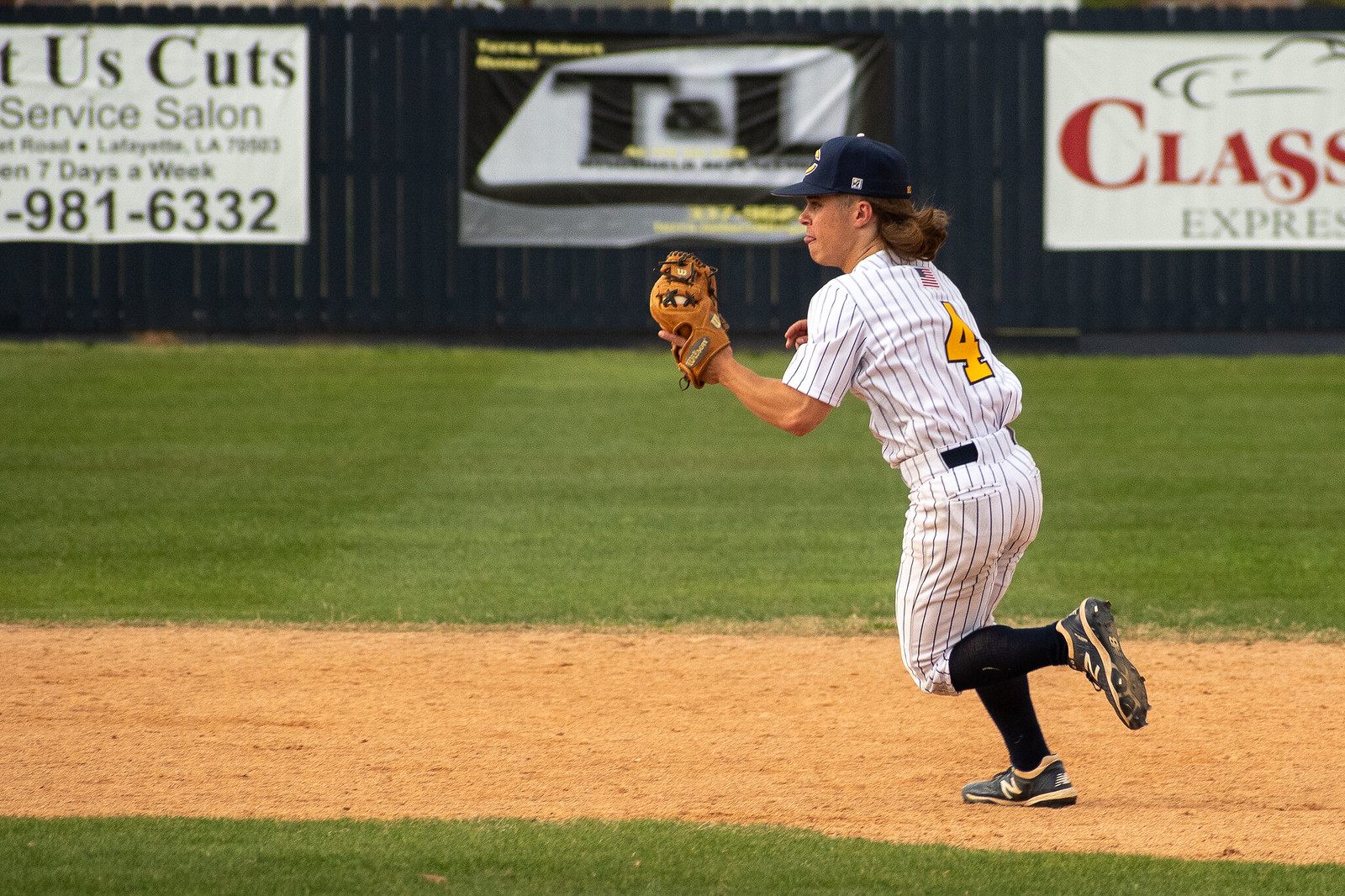The image depicts a baseball game featuring a young athlete, possibly in their early teens or late elementary school years, wearing a pinstriped white uniform with a black belt, socks, and New Balance cleats. The player, with "New Balance" cleats and the number "4" in yellow with a black outline on their back, is running across the infield dirt with their left foot in the air and a glove on their left hand. A flag is displayed above the number on their back. The player seems to be either catching a ball or preparing to catch one. Surrounding the field is a blue fence adorned with various advertisements, including those for a full-service hair salon and a company called "Glass Express". Partly visible text on one ad suggests it serves the Lafayette, LA area and operates seven days a week.